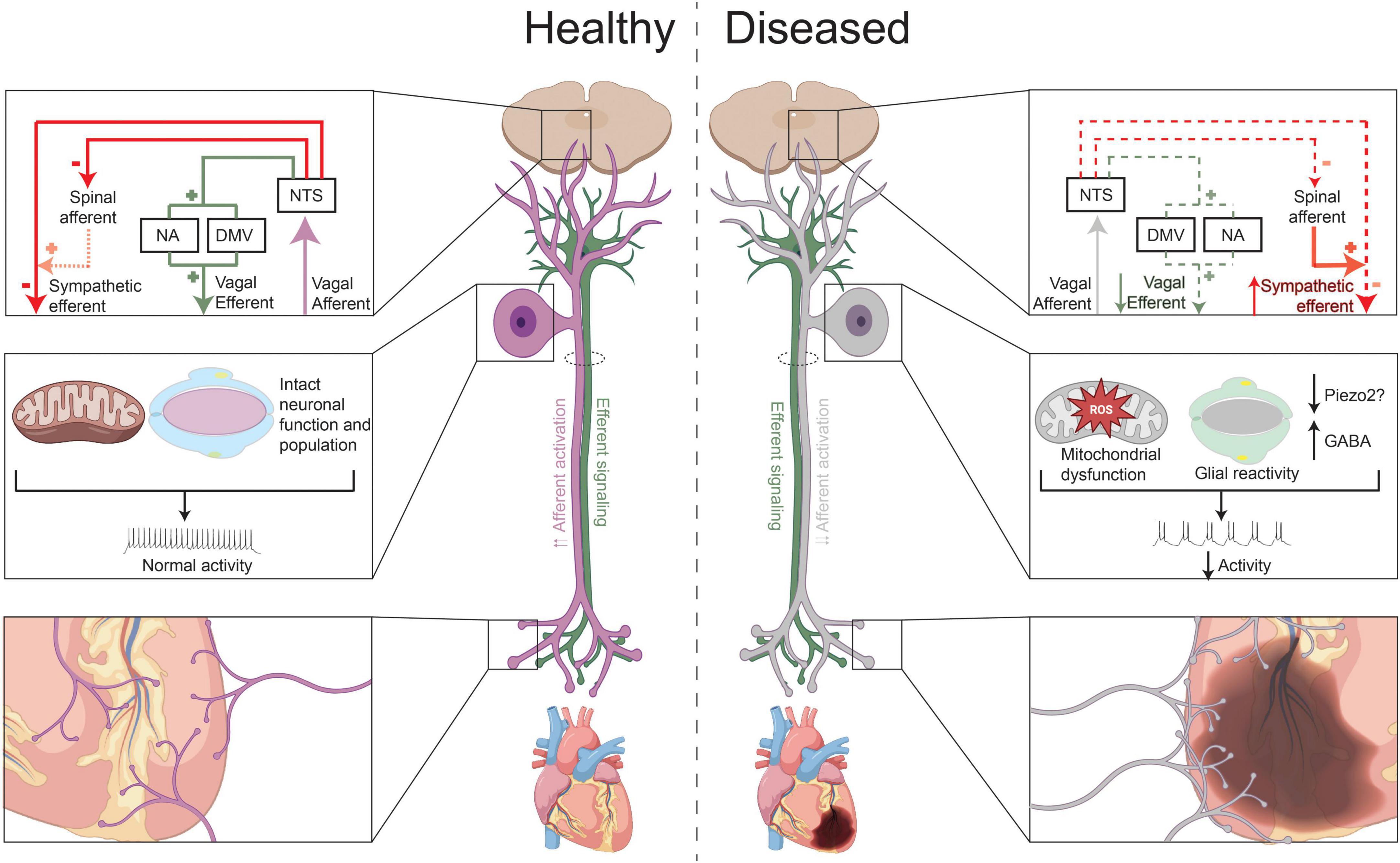The image, set against a solid white background, features two side-by-side diagrams. The left diagram is labeled "healthy" and the right diagram is labeled "diseased." Both diagrams depict the same biological system, illustrating a plant stem alongside representations of the brainstem and heart. 

The "healthy" side prominently features a purple color scheme, with diagrams and arrows indicating various healthy conditions and interactions extending from the brain to the heart. Detailed sections zoom into specific areas, providing further insights into the well-functioning system.

In contrast, the "diseased" side uses a blue color scheme to delineate the pathological state of the same system. Various diagrams, figures, and arrows highlight key areas of concern, illustrating how the disease impacts the plant stem, brainstem, and heart.

Overall, the composite illustration uses flowcharts, detailed figures, and magnified insets to compare and contrast the healthy and diseased states of the biological system, emphasizing the transition from normal function to pathology.